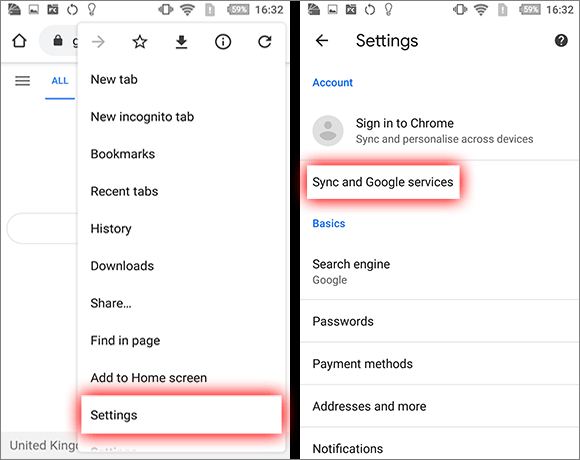The image displays a split-screen view. On the left side, there's a website interface featuring a search bar at the top, followed by black menu bars. The word "All" is highlighted in blue. A pop-up menu is layered over the webpage, showing several icons and text options, listed as follows: an arrow pointing right, an outline of a star, a thick arrow pointing down, a circle with an eye in the center, and another circle with an arrow. The menu items are "New tab," "New incognito tab," "Bookmarks," "Recent tabs," "History," "Download," "Share," "Find in page," "Add to home screen," and then "Settings," which is highlighted with a red outline. The word "United Kingdom" is partially visible below this menu, next to a thick vertical black line.

On the right side of the screen, the "Settings" page is shown. The title "Settings" is in black with an arrow pointing left, accompanied by a white question mark inside a circle. The section titled "Account" is in blue, featuring a gray circle with a person icon, and below it reads "Sign in to Chrome - sync and personalize across devices." "Sync in Google services" is highlighted in red. Below it, the "Basics" section is in blue, listing "Search engine: Google," "Passwords," "Payment methods," "Addresses and more," and "Notifications," each separated by fine lines.

At the top of both screens, common status icons are visible: the time "16:32," a battery icon at 59%, a cell phone signal icon, volume bars, and a gray square with an exclamation point. On the left side of each page, there are five small icons whose meanings are unclear: a light bulb, two arrows forming a circle, a black box with "FC," a gray box with dots, and a half-circle icon.